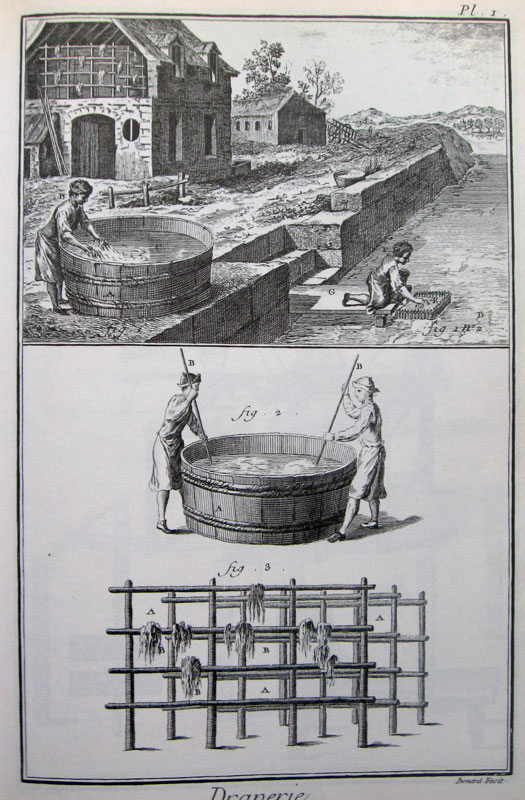The image is a vintage black-and-white drawing, possibly created with black ink or pencil, capturing two distinct scenes on a rectangular, gray-toned piece of paper. The top half of the graphic showcases an old, large brick barn with a block wall perimeter, nestled amid various buildings, including one with numerous windows. In the foreground, a mother figure is bent over a sizable wash tub, diligently washing clothes, while a child plays nearby, adding a touch of everyday life to the serene countryside landscape. Leading from the wash area, a set of stairs descends to a riverbank where another individual is engaged in a separate activity—possibly fishing or dyeing textiles—connecting the rural homestead to the waterway.

In the bottom half of the image, the focus shifts to a more detailed depiction of the washing process. Two people stand on either side of a large wooden vat or bin, stirring clothes with long sticks. Below this scene, there is a diagram featuring a crosshatched wooden clothes hanger, resembling a tic-tac-toe grid, adorned with clothing items, perhaps drying or being aired out. Additional fence posts with rags hanging suggest an expanded area for drying fabrics. This lower segment illustrates the traditional methods of washing and drying clothes, emphasizing the labor-intensive practices of the past.